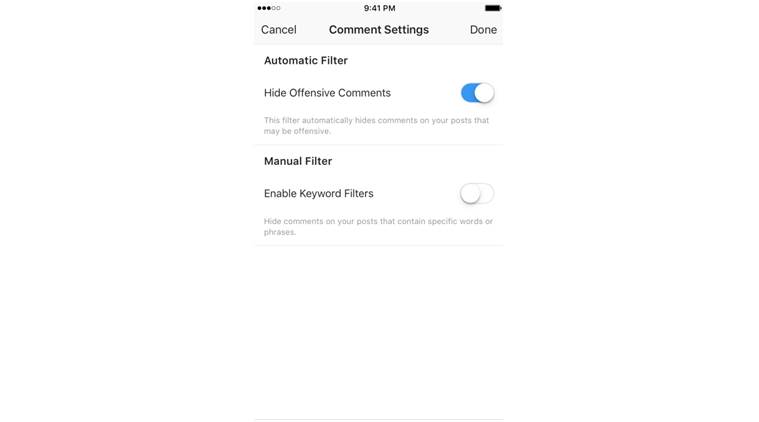This image is a screenshot taken from a cell phone at 9:41 p.m., as indicated by the digital clock at the top of the screen. The status bar shows five horizontal dots, three of which are filled in black while the remaining two are gray. Additionally, the battery icon at the far-right end of the status bar is completely filled in black, suggesting that the battery is fully charged.

Below the status bar, the interface features a Cancel button on the left and a Done button on the right, flanking the title "Comment Settings". 

In the main content area, the first section is titled "Automatic Filter". Under this section, there is an option labeled "Hide Offensive Comments" that is currently enabled, as indicated by a blue slider bar with a white circle on the right.

Further down, the "Manual Filter" section includes an option for "Enable Keyword Filter", which is presently disabled. This is shown by a fully white slider bar with a white circle on the left. A description below explains that enabling this feature would hide comments on your posts that contain specific words or phrases.